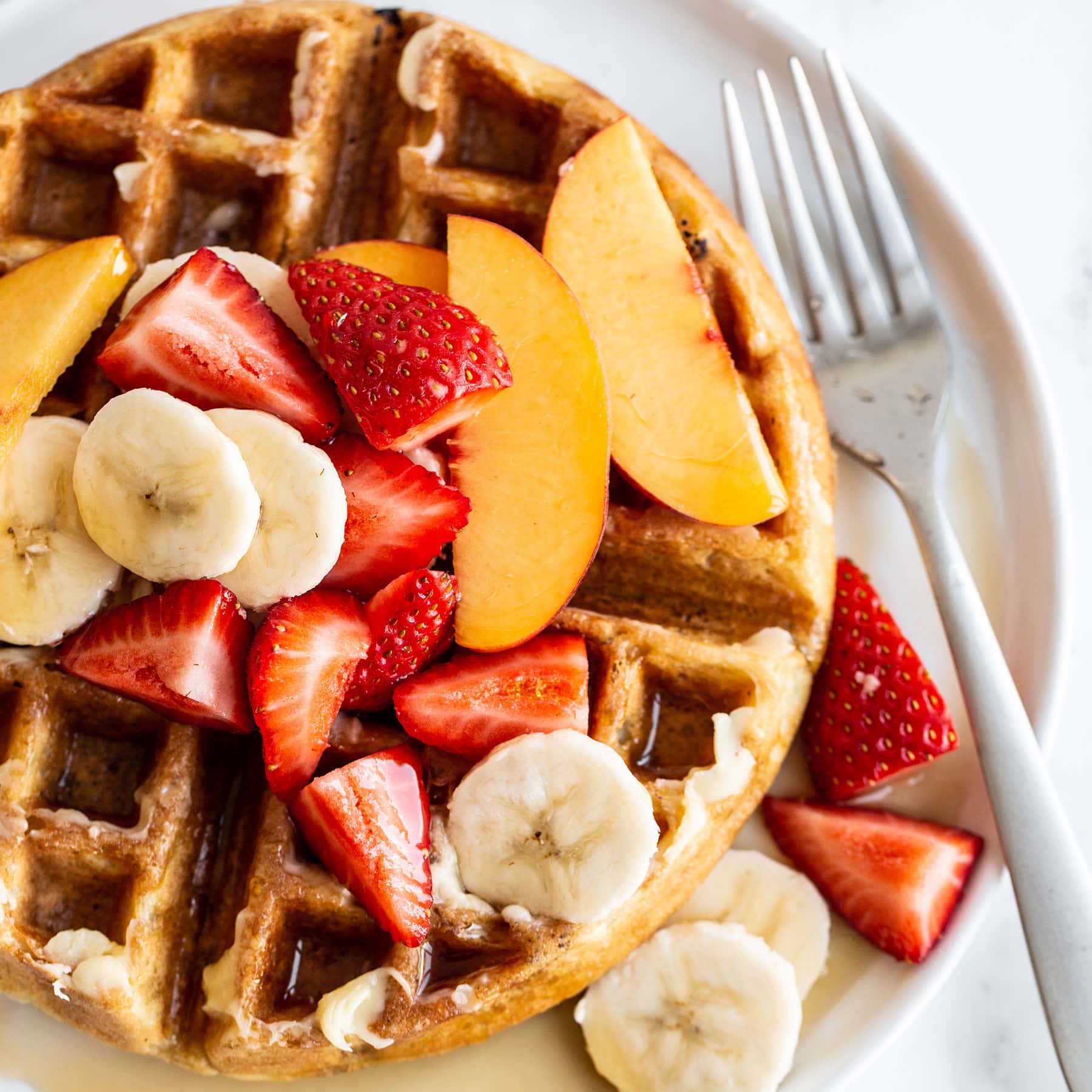This close-up, professional image captures an appetizing breakfast plate set against a white, marble-like background. Centered on a pristine, white dish is a golden brown, round Belgian waffle divided into four quarters. The waffle is generously topped with glistening syrup, a dollop of unmelted butter, and an assortment of fresh fruit. Prominently featured are bright red strawberries sliced into spear shapes, circular banana slices, and crescent-shaped peach slices. Nearby, two banana slices and two strawberry slices have slipped off the waffle and rest beside a silver fork positioned to the right of the plate. The inviting composition highlights the contrasting colors and textures of the fruits against the waffle, making it an enticing start to the day.